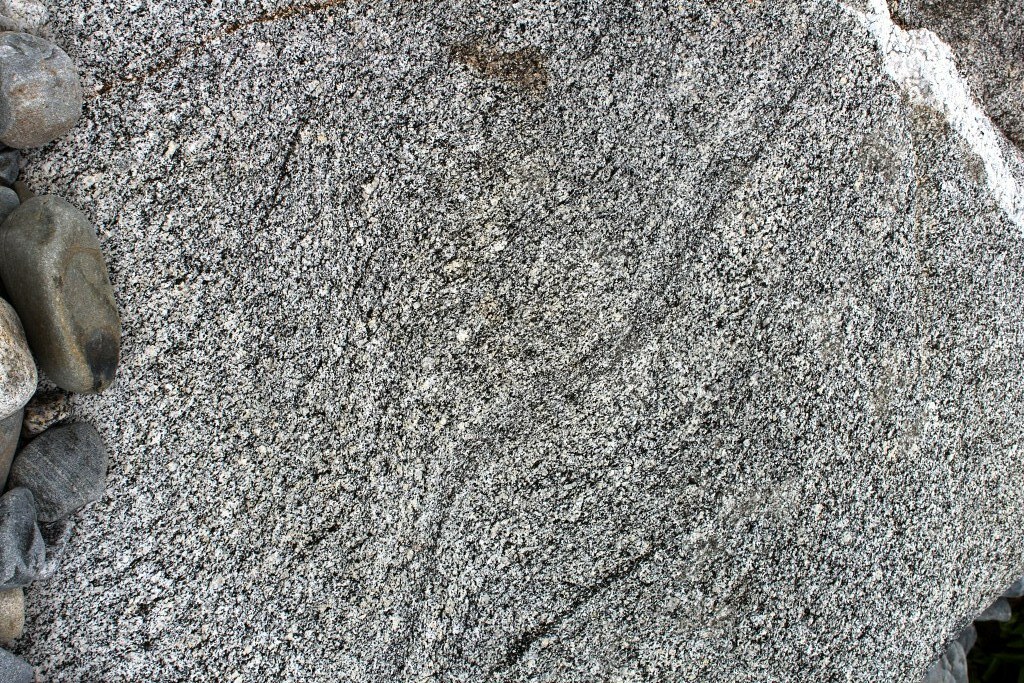The image depicts a close-up view of an outdoor scene centered on a large, flat slab of slate-like stone, characterized by its intricate and varied coloration ranging from gray and white to black and brown. The stone has a rough texture and includes some distinct brownish spots and dark stains. On the left side of the image, there is a collection of smaller, smoother stones in shades of brown, black, white, gray, and slate. These stones appear intentionally placed and provide a stark contrast in texture and color to the larger slab. The photo is likely taken during daylight, given the natural lighting and outdoor elements, with the camera positioned directly above, capturing a detailed and focused perspective of the main stone and its surroundings.